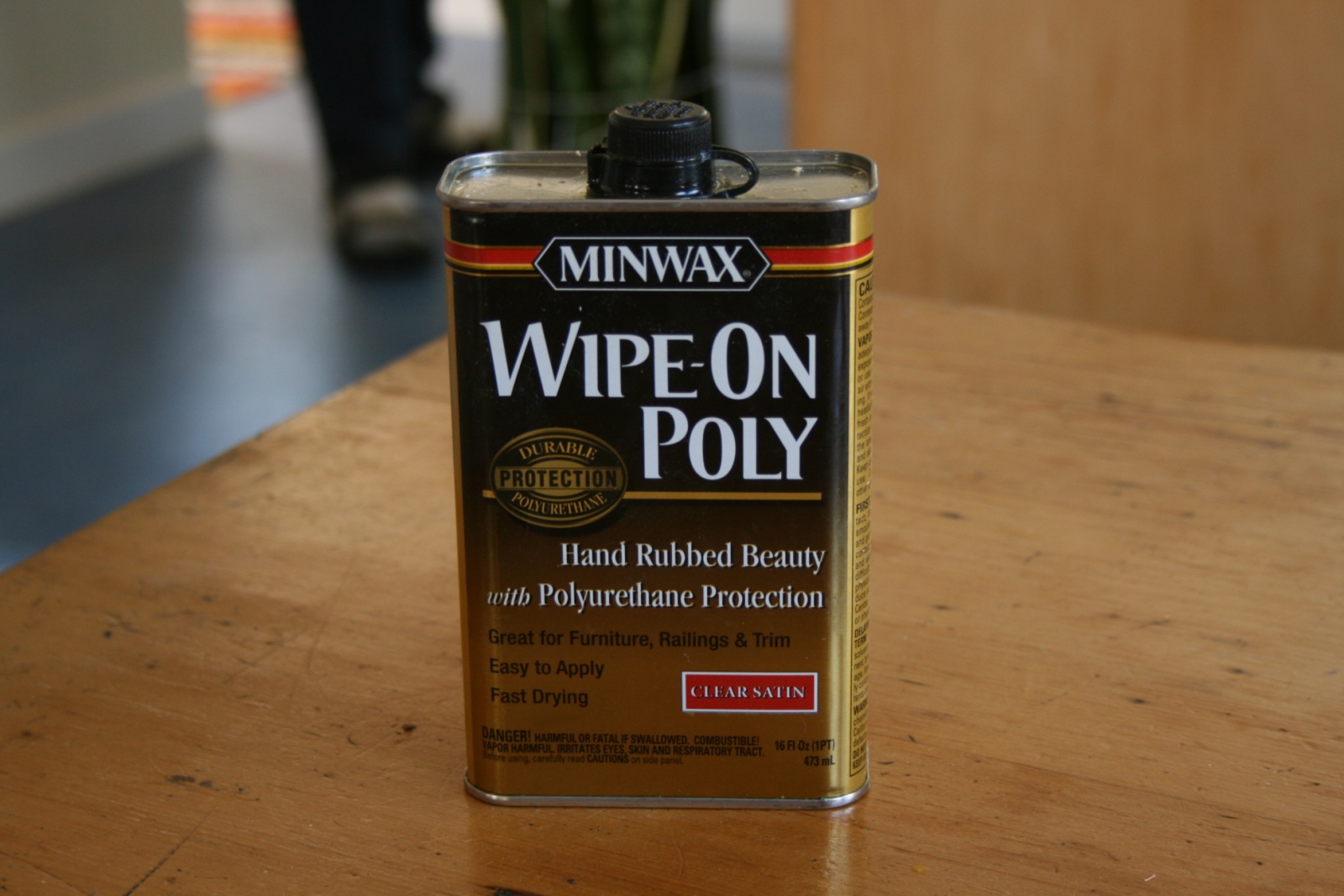The image depicts a close-up of a canister of "Wipe-On Poly," a product by Minwax. The container is primarily gold with distinctive red striping around it, and it features a black cap at the top. The front label reads "hand-rubbed beauty with polyurethane protection" and emphasizes its promise of "durable protection." The detailed label and color scheme make the product easily recognizable as a high-quality, versatile wood finish.